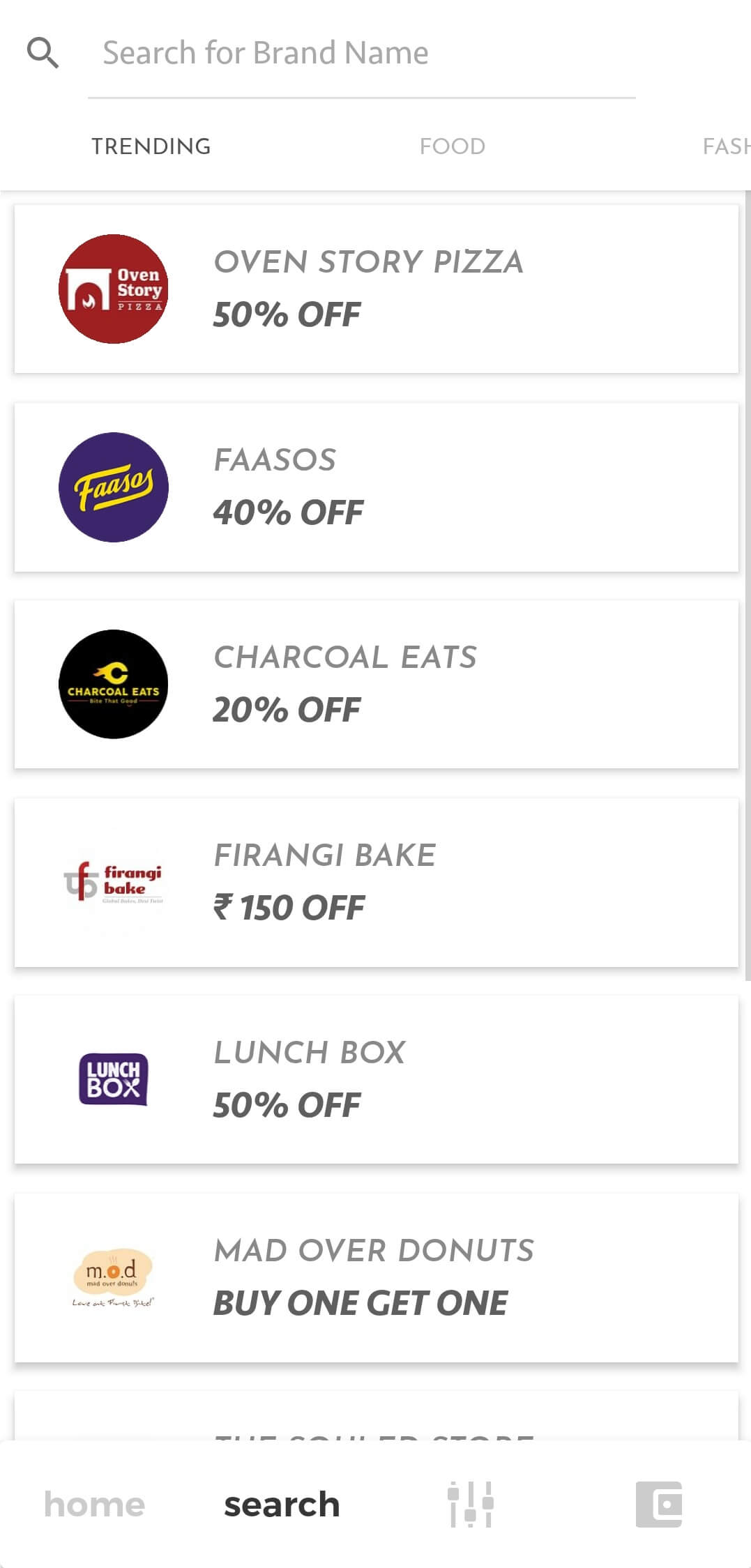The image is a vertically oriented screenshot from a smart device, featuring a white background that looks to be derived from the user's computer screen. At the top left, there's a magnifying glass icon followed by the text "Search for brand name." Below this, a gray separator line divides the search bar from various selection options. The "Trending" tab is currently selected, while other partially visible options include "Food" and the beginning of a word that might be "fashion."

Beneath these tabs, several horizontal boxes span across the screen, each containing an image and text. The first box promotes "Oven Story Pizza" with a 50% discount. Next is "Faasos" offering 40% off, followed by "Charcoal Eats" with a 20% discount. Each promotional box is enclosed in a gray border and set against the white background.

Further down, another box features "Ferrangi Bake," which offers a discount of 150 units of an unspecified currency. Following this is "Lunchbox" with a 50% discount, and "Mad Over Donuts," which offers a "Buy One, Get One" deal. A partially visible box at the bottom suggests there is one more promotion not entirely captured in the screenshot.

At the very bottom of the image, the device's home button is visible, along with a highlighted search icon and several other navigation icons.